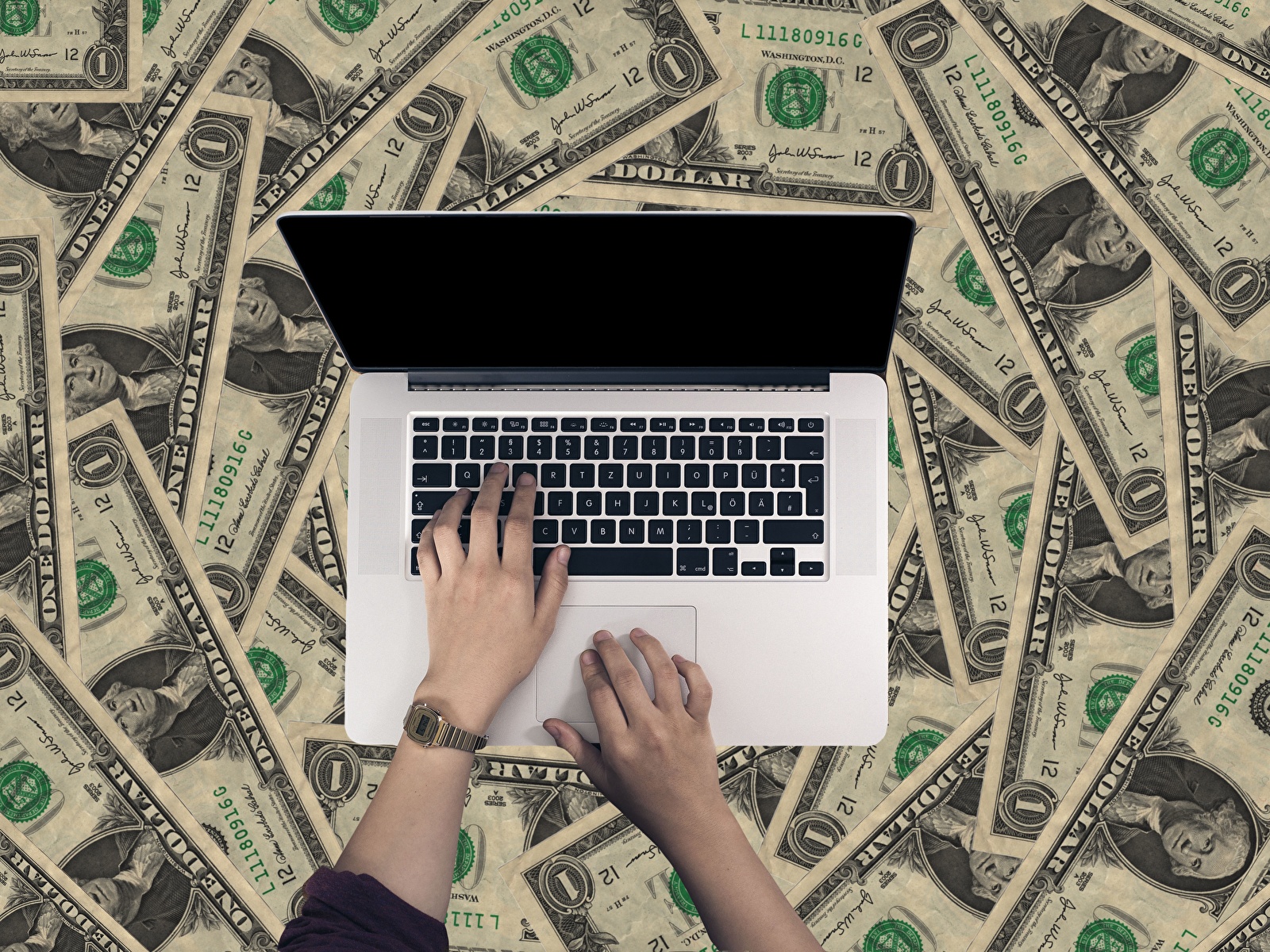This composite photographic illustration shows an overhead view of a whitish laptop with a black keyboard, set against a background meticulously crafted from layered one-dollar bills. The laptop screen appears black and gives an impression of being blank. Two hands are actively engaged with the laptop: the left hand, adorned with an older digital watch and partially covered by a pushed-up sleeve, types on the keyboard in the region commonly associated with the WASD keys. The right hand operates the touchpad. The background dollar bills, all single one-dollar notes, feature varying angles and overlap each other in a decoupage-like style, creating a textured mosaic of currency. The distinctive visage of George Washington on each bill and the prominent numerals "1" mark these as unmistakably American one-dollar bills. Although there's a mention of differing skin tones implying that the hands might belong to two different individuals, the overall composition focuses on the unified activity of interacting with the laptop amidst a cascade of money.